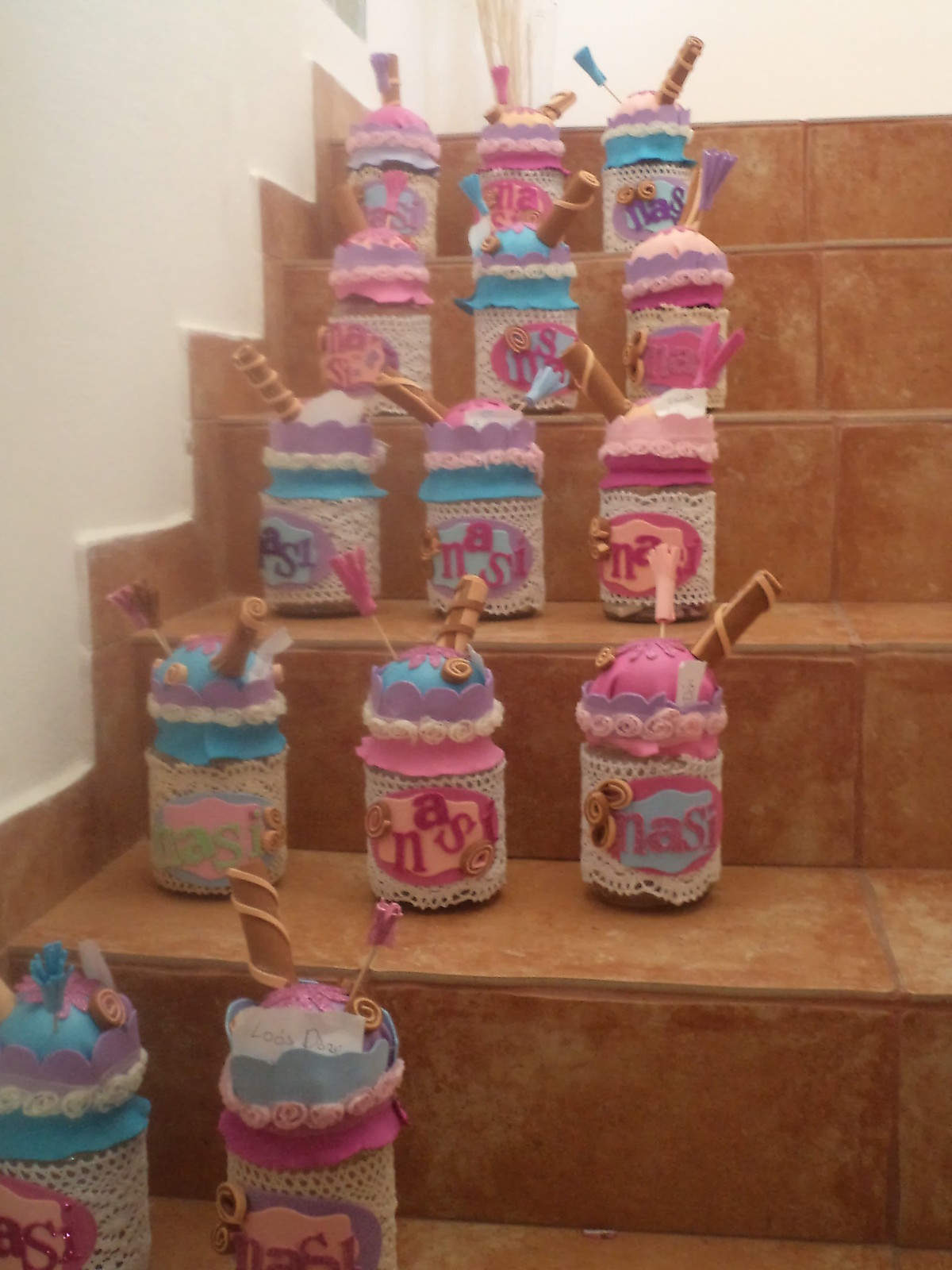This image showcases a craft project displayed on a rustic, terracotta-tiled stairway. On each step of the stairway, there are decorated canisters arranged in rows, predominantly towards the left side as one ascends. The canisters, fourteen in total, are embellished with cream-colored doilies wrapped around their bodies. Each canister features a front label that spells out "NAS" and is topped with a lid covered in felt, adorned with tiny roses and a ripple-like crown effect. Some lids are pink, and others are blue or purple, adding a playful, birthday cake-like appearance. Additionally, each canister has a stick of cinnamon protruding from the felt lid, giving them a whimsical touch. This meticulously detailed display appears to be a charming craft project, perhaps created by children, that blends various textures, colors, and decorative elements into a cohesive and eye-catching arrangement on the staircase.